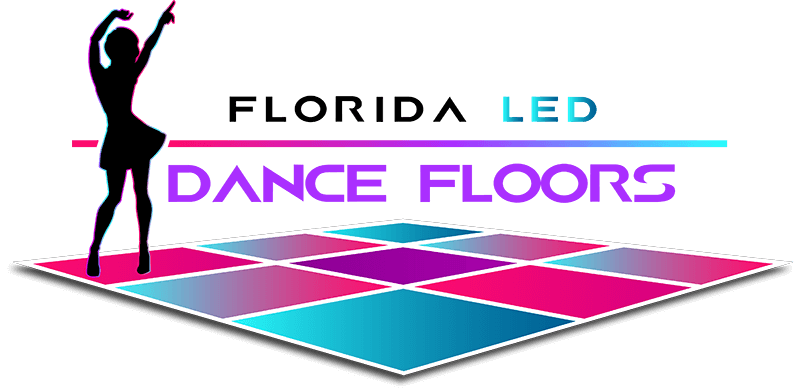This image is a digitally generated advertisement for a company specializing in dance floors, prominently featuring the company name "Florida LED Dance Floors." The background is pure white, and the image is horizontally rectangular without a border. Central to the design is the logo: "Florida" in black text, with the 'A' represented creatively as an upside-down 'V'. Below it, "LED" appears in a gradient of blue shades, transitioning from light blue to a darker blue on the right. The words "Dance Floors" are displayed in dark purple.

Adjacent to this logo, on the left side, is a silhouette of a woman in a very short skirt, outlined in pink and neon green. She is depicted dancing with her hands up in the air and one hip kicked out. Beneath the text, there is an illustrated dance floor composed of a grid of colored squares - blue, red, pink, and purple - segmented by vertical and horizontal white lines. The woman is positioned on a pink square, creating a vibrant focal point that complements the multi-colored, checkered dance floor.